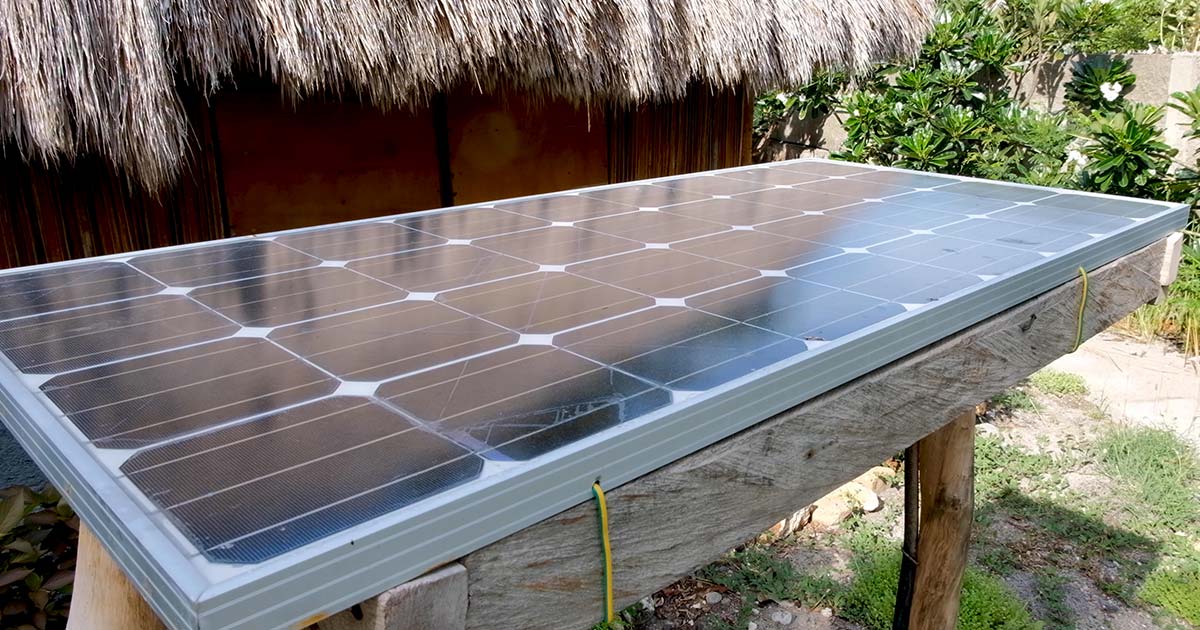This outdoor photograph features a solar panel with a distinctive checkerboard design, outlined in white and with black squares, mounted on a wooden table-like structure resembling a saw horse with light brown legs. Yellow cables extend from the right side of the panel, connecting it to the wooden base. Behind the solar panel, on the left side, stands a brown hut with a tan, thatched roof, reminiscent of a tiki or palapa structure. To the right, a gray stone wall adorned with various green plants, displaying both dark and light green leaves, adds a natural backdrop. The ground below comprises a mix of green grass, light brown dirt, and stone, interspersed with a white walkway that runs in front of the wall. The overall scene captures a harmonious blend of man-made and natural elements in a rustic setting.